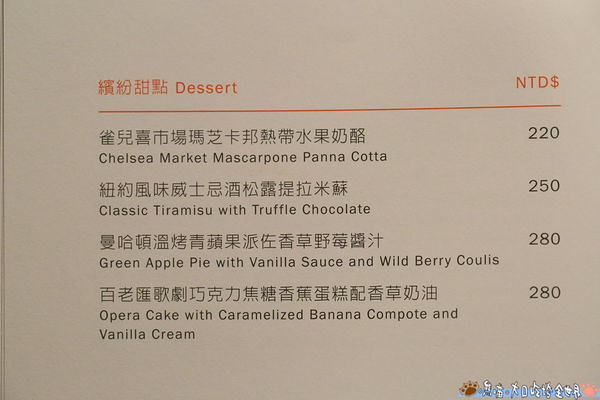The image depicts a menu on a gray cardstock, featuring four dessert items listed in both English and what appears to be Asian, possibly Chinese, characters. At the top left, there are some Asian symbols followed by the word "Dessert" in red text. On the far right, the letters "NTD" followed by a dollar sign are highlighted in orange. Below this, a thin orange line separates the header from the dessert listings. The desserts are presented in black text, each preceded by Asian characters and accompanied by their respective prices in NTD dollars. The items are Chelsea Market Mascarpone Panna Cotta for $220, Classic Tiramisu with Truffle Chocolate for $250, Green Apple Pie with Vanilla Sauce and Wild Berries for $280, and Opera Cake with Caramelized Banana Compote and Vanilla Cream for $280. In the bottom right corner, further Asian symbols are displayed.